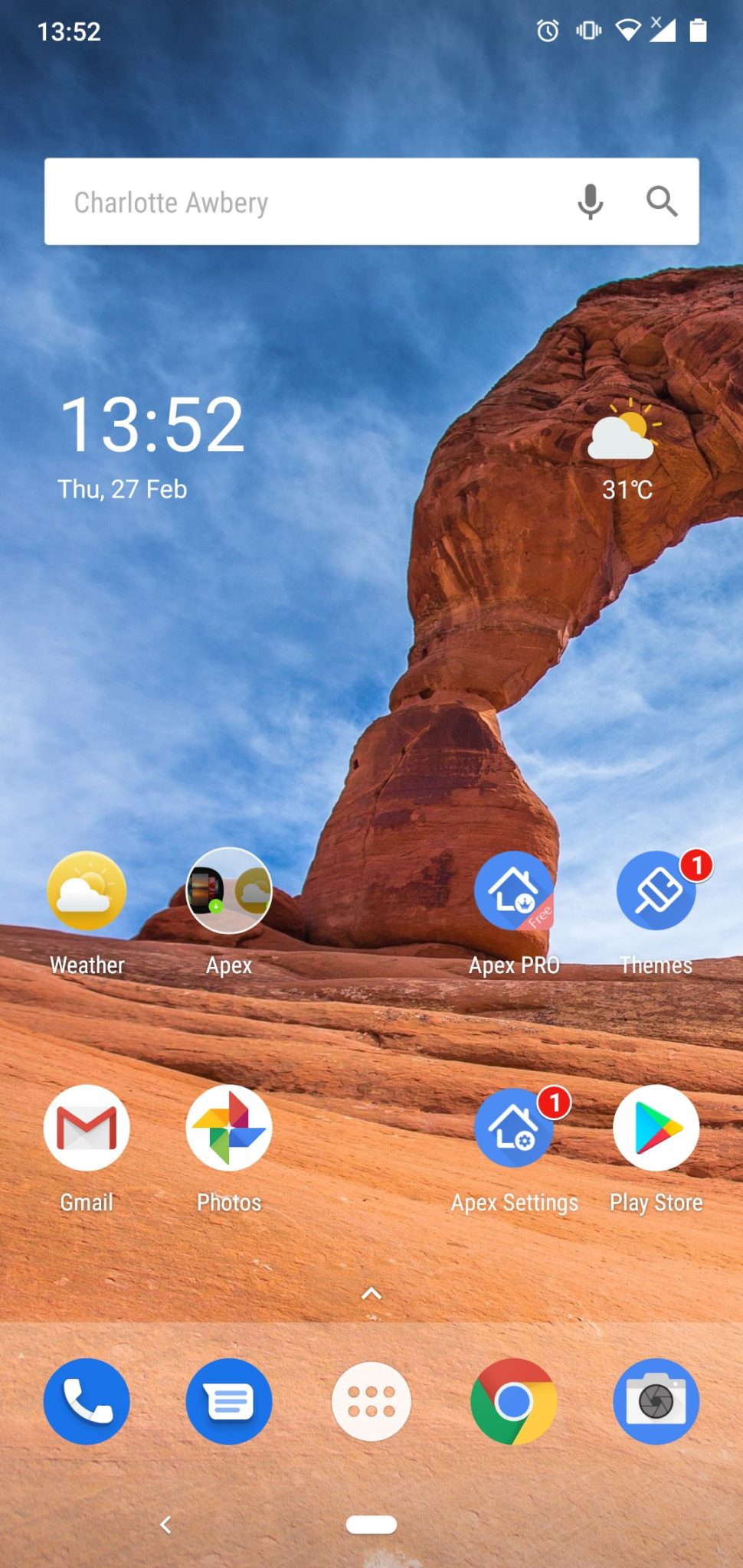The image is a detailed screenshot of a smartphone displaying its home screen. The background photograph depicts a serene desert landscape with a vibrant blue sky, accentuated by a striking rock formation. In the upper left corner of the screen, the current time is displayed prominently. Adjacent to it on the top right are various status icons indicating battery life, Wi-Fi connectivity, and other essential notifications. Below this, there is a search bar widget designed for quick, on-screen searches. The main section of the screen is populated with a series of application icons, which include commonly used apps such as Weather, Photos, Chrome, Play Store, and Phone. Each icon is neatly arranged, reflecting the typical layout you would expect to find on a well-organized smartphone interface.